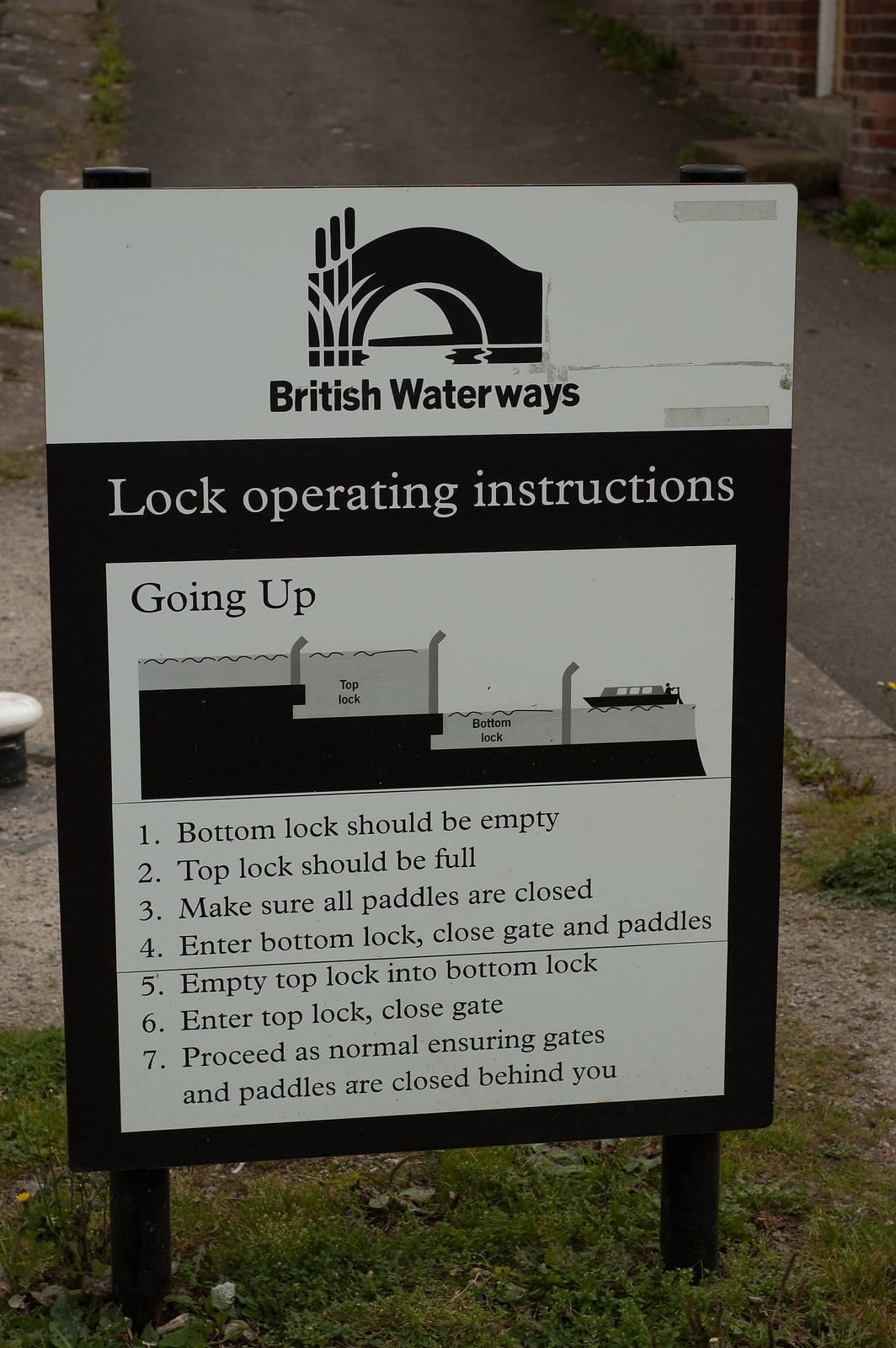The image prominently features an informational signboard positioned alongside an asphalt pathway, surrounded by a patchwork of grass, dirt, and gravel. The signboard is supported by two sturdy black poles. At the very top of the signboard, there is a white-bordered section displaying a stylized logo of a bridge and the text "British Waterways" in bold black font.

The main body of the sign has a black background, with the heading "Lock Operating Instructions" at the top in white text. Below this heading, a white rectangular graphic illustrates several river locks and demonstrates their operation. Detailed step-by-step instructions are listed underneath:

1. Bottom lock should be empty.
2. Top lock should be full.
3. Make sure all paddles are closed.
4. Enter the bottom lock, close gate, and paddles.

The instructional content is clear and well-organized, designed to guide users through the lock operation process efficiently.